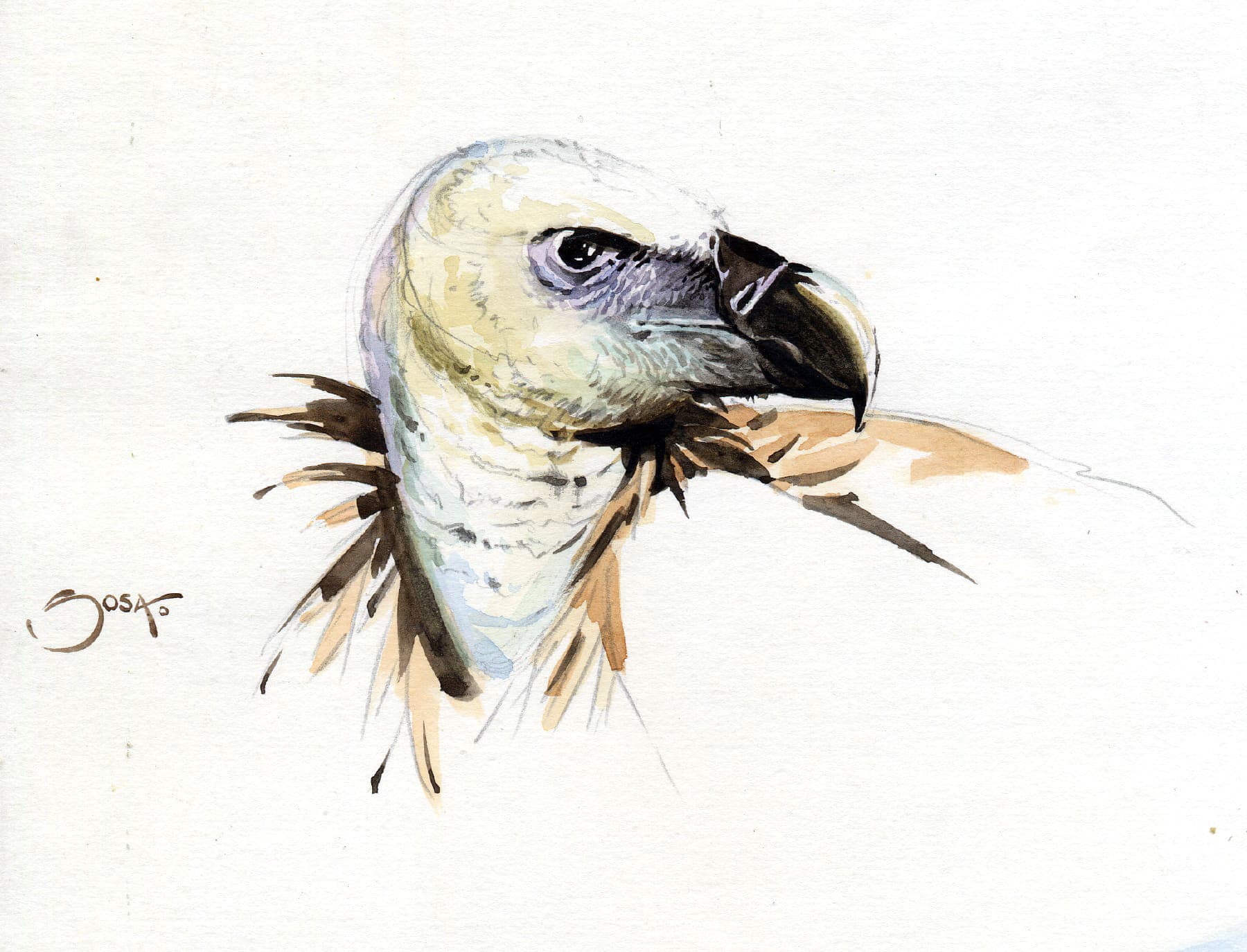On a stark white background, this artistic drawing focuses on the head and neck of a bird, featuring a detailed mix of colors and textures. The bird's head, predominantly white with some tan and gray spots, turns to the right, exposing a sharply pointed, black hook-like beak. Around the eyes, tinged with purple and hints of yellow, it creates an intense, predatory gaze. Brown and pink feathers adorn the upper neck and top of the head, transitioning into lighter, sketchy lines that hint at an unfinished rendering beneath the neck. Below, to the left, lies the artist's signature "SOSA" in brown, accompanied by a small "D".